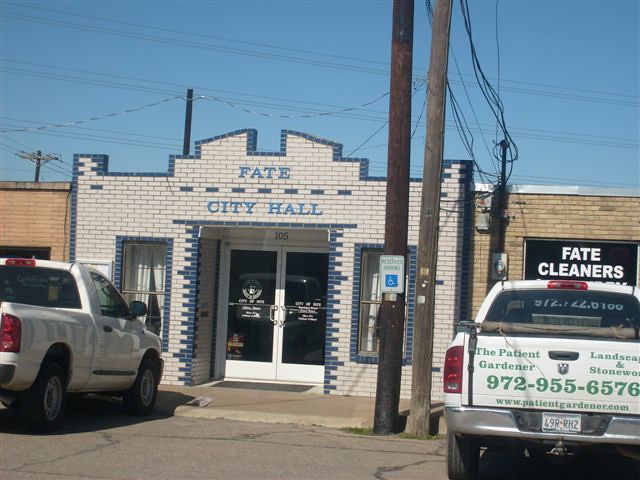Set against a clear blue sky, this outdoor photo depicts a quaint, single-story building in what appears to be a small town. The structure is characterized by white brickwork with blue trim, featuring a notable archway above two glass doors. These doors have an arch resembling a piano keyboard in alternating blue and white bricks, adding a unique charm. Inscribed in bold blue letters above the entrance is "FATE City Hall," indicating the building's purpose.

Adjacent to the City Hall is another business, Fate Cleaners, with its name displayed prominently in white letters on the window. Two white pickup trucks are parked in front: one is partially visible, while the other, stationed near Fate Cleaners, portrays "The Patient Gardener Landscaping and Stone Work" on its rear with a contact number underneath. The scene is completed by a handicapped parking sign on a pole near the entrance, adding a touch of everyday practicality to the picturesque setting.